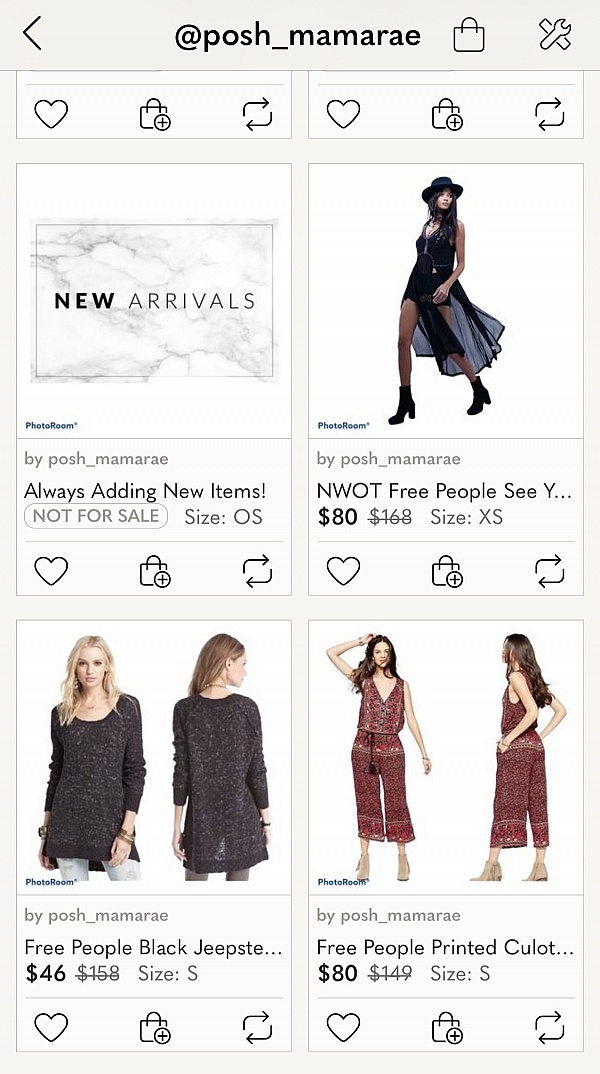This is a detailed description of a screenshot from a product listing page on a mobile application. The background is beige, including the header, which is distinguished by a light gray underline. On the left of the header, a dark gray arrow points left, indicating a back navigation option. Centered in the header is black text displaying the username "@posh_mamaray." To its right, there is a shopping bag icon followed by a crossed ruler and wrench icon.

The body of the page maintains the beige background. Each product is displayed within a vertical rectangular tab, featuring a white background with a photograph at the top. Below the photograph is a gray section containing light gray text that credits the seller, "@posh_mamaray." This section also includes the product title in black text, additional information, and, after a thin gray line, three icons: a heart, a shopping bag with a plus sign encircled, and a refresh icon represented by two black arrows (one pointing right and one left). 

Products are displayed two per row vertically. Moving through the items, a photograph of a marble countertop labeled "New Arrivals" is shown. To its right, there's a photograph of a woman in a flowing black dress wearing a black hat, accompanied by the text "NWOT Free People C..." in bold black text displaying "$80," with the original price of "$168" crossed out in light gray and the size "Extra Small" in light gray.

Beneath this row, the next items listed are "Free People Black Jeepster..." and "Free People Printed Kula..."